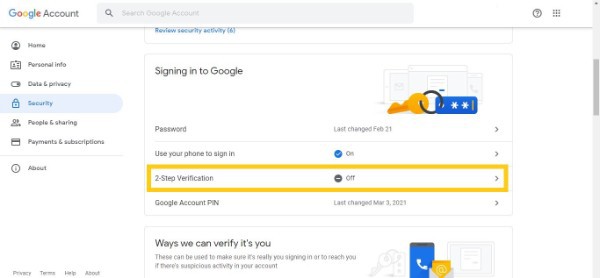The image is a left-to-right, horizontal screenshot, seemingly captured from a computer or smartphone device. The interface predominantly features elements from a Google Account settings page and appears to borrow a portion of the white background typical of such applications.

At the top left, the text "Google Account" is prominently displayed, accompanied by a rounded, elongated, gray rectangular search bar labeled "Search Google Account." Directly below this header, a vertical menu presents several options: Home, Personal Info, Data and Privacy, Security (highlighted), People and Sharing, Payments and Subscriptions, each prefaced by a respective icon. A separating line below this menu introduces the About section, and further down at the bottom left, additional options such as Privacy, Terms, Help, and About are visible.

On the upper right, a small question mark icon within a circle and a grid icon provide quick navigation tools. Centrally, the blue text "Review Security Activity" is conspicuously positioned with a notation of "(6)" indicating available actions or alerts. Below, a black heading, "Signing in to Google," leads to detailed security settings, including:

- **Password**: Information on the last change.
- **Use your phone to sign in**: Featuring an active toggle.
- **Two-step verification**: Highlighted with a prominent long orange box, currently turned off.
- **Google Account PIN**: Denotation of its last change in March 2021.
- **Verification methods**: Various icons and options for user verification.

The right-hand border of the screen includes a vertical gray scrollbar designed for navigating the page content up or down.